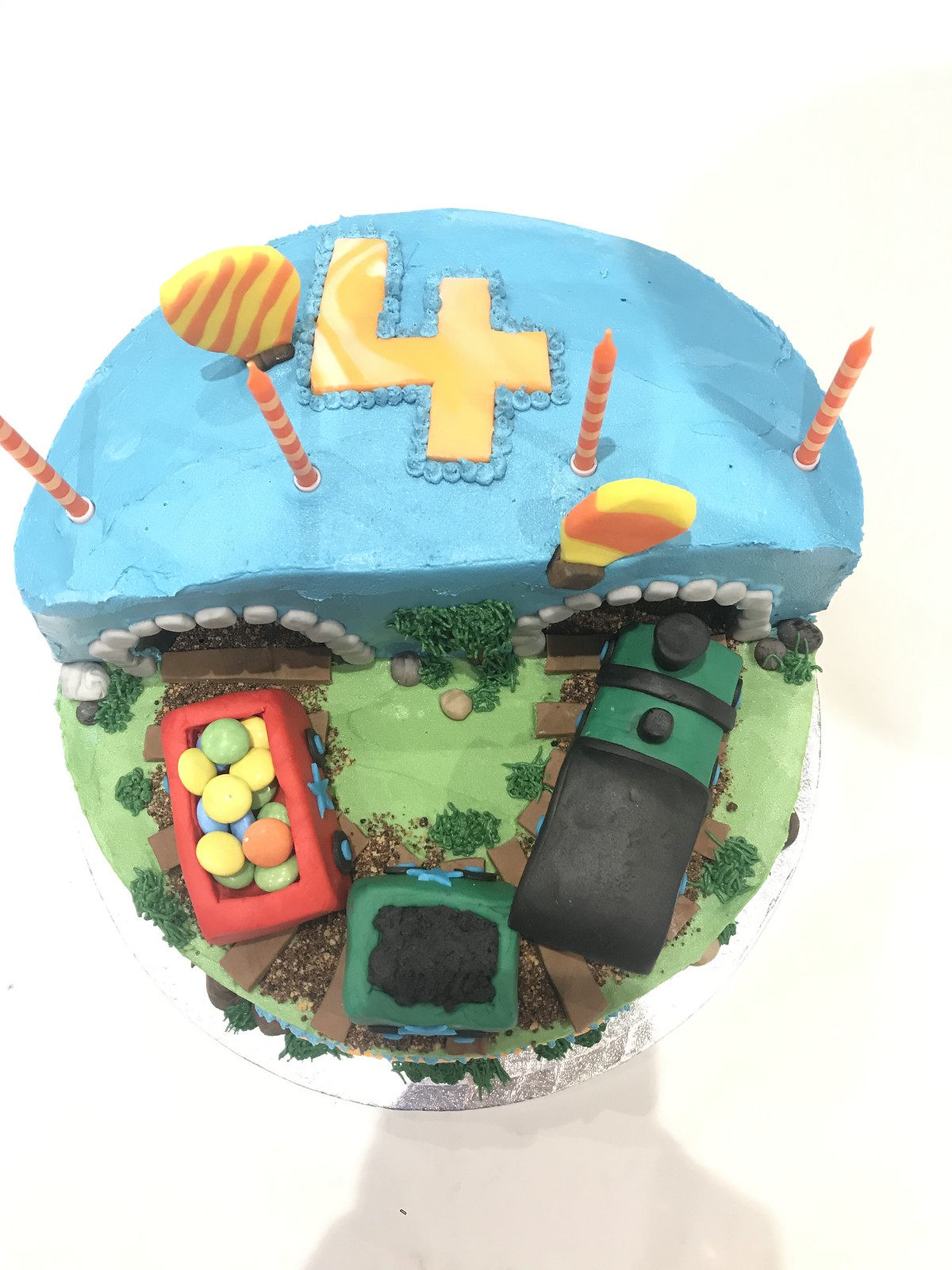This image captures a detailed, multi-tiered birthday cake designed to resemble a whimsical train scene. The cake is set against a white background and sits on a silver or white paper plate base. The top half of the cake is elevated, covered in blue icing, and adorned with four orange and white spiral candles and an orange number four with blue dots lining its border. This elevated section appears as a cave or tunnel entrance for a train below. The lower half of the cake, about three inches lower, features green icing textured to look like grass with patches of darker green. Here, a train engine leads a coal car and a second car filled with colorful candies resembling M&Ms (yellow, green, blue, and orange) along a track. The scene is further detailed with small plants, rocks, and two tiny hot air balloons in the sky, creating an ornate and imaginative birthday display.